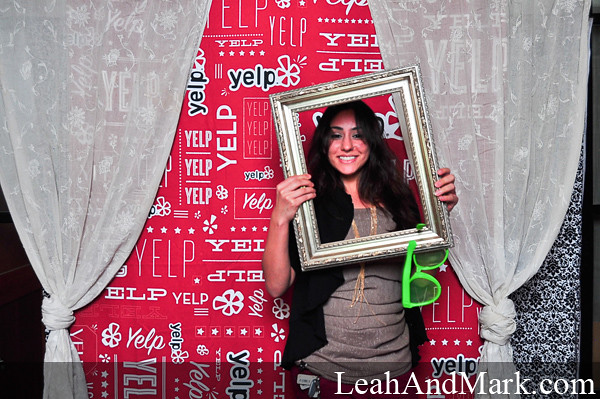In this vibrant color image, a young woman stands smiling in front of a red background emblazoned repeatedly with the word "Yelp," suggesting a promotional event for the website Yelp. The red backdrop is flanked by sheer white curtains tied near the bottom, adding a touch of elegance. The woman holds an antique picture frame around her head and shoulders, giving the illusion that her face is being framed. Dangling from the bottom of the frame is a large pair of oversized green sunglasses, adding a playful element to the scene. She has long black hair, wears a gold necklace, and is dressed in a gray shirt with a black vest-like coat. The artistic setup is further marked with a web address, "leahandmark.com," located in the bottom right corner, hinting at possible photography credits. Additionally, behind the red Yelp background, another layer of a white and black backdrop is visible, enhancing the depth and complexity of the scene.